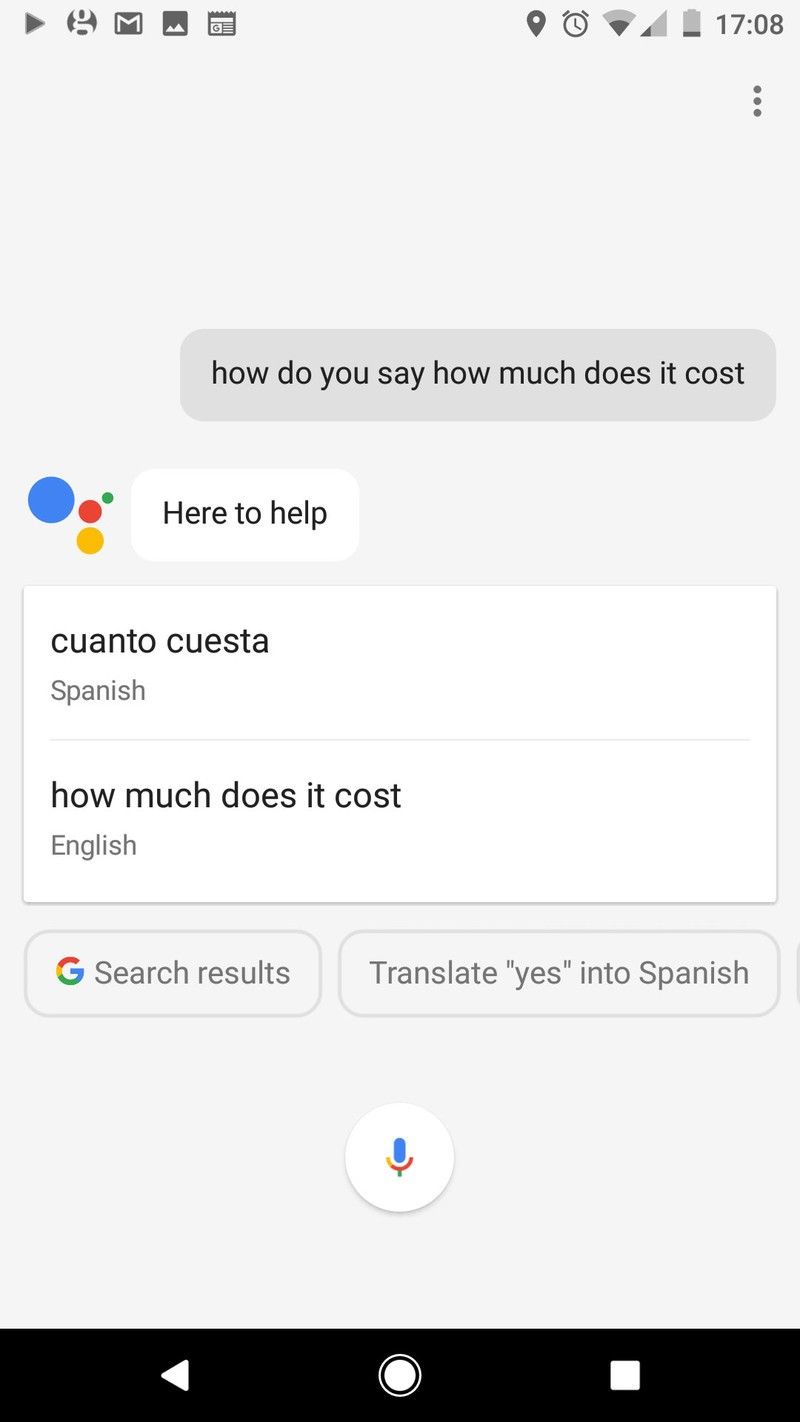The image is a screenshot of a smartphone screen. In the top-left corner, there is a collection of icons: a play button, a key resembling the Google symbol, the Gmail icon, a picture symbol, and an icon that appears to be a certificate with a key on it. On the far right, there are symbols indicating location, an alarm, Wi-Fi, cellular signal, and a battery icon showing low battery. The time displayed is 17:08, and below the time are three vertical dots. 

Underneath this, a Google search has been initiated with the query, "How do you say how much does it cost?" The search result page features the Google logo with the text "Here to help." The top results are "¿Cuánto cuesta?" in Spanish, followed by "How much does it cost?" in English. There are two buttons below these translations: one reads "Key search results," and the other says "Translate 'How much does it cost?' into Spanish."

At the bottom of the screen, there is a white circle with the Google search icon in the center. Below this are the smartphone navigation buttons: a back button on the left, a home button in the center featuring a white button with a black and white border, and a recent apps button on the right depicted as a white square.